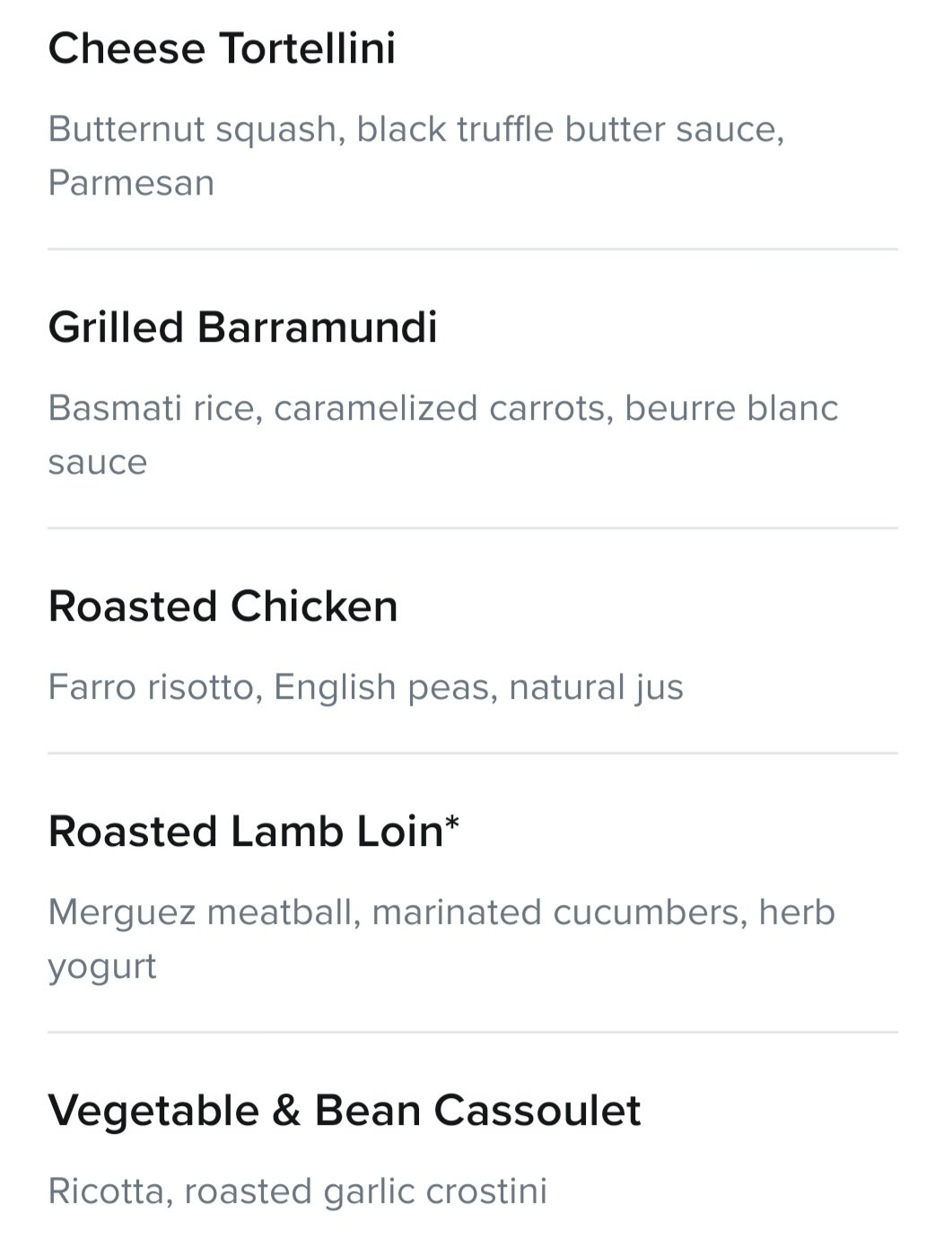Below is a cleaned-up and detailed descriptive caption for the provided menu image:

---

The image displays a restaurant menu on an app, potentially DoorDash, with several delectable offerings:

1. At the top left, the dish 'Cheese Tortellini' is prominently displayed in black font. Below this, in smaller gray font, it lists the ingredients: 'Butternut Squash, Black Truffle Butter Sauce, Parmesan.'
2. Beneath this section, there is a gray line divider, followed by the next dish: 'Grilled Barramundi' written in bold black font. Underneath, in smaller gray letters, the detailed components are noted: 'Basmati Rice, Caramelized Carrots, Beurre Blanc Sauce.'
3. Another divider separates the subsequent item, 'Roasted Chicken,' marked in larger black font. Described in light gray below, the dish includes: 'Fara Risotto, English Peas, Natural Jus' (with a portion of the description abbreviated).
4. Following another divider is the 'Roasted Lamb Loin,' highlighted in big black lettering with an asterisk. The description, in smaller gray font, reads: 'Merguez Meatball, Marinated Cucumbers, Herb Yogurt.'
5. The last listed entrée separated by another gray line is 'Vegetable & Bean Cassoulet,' with 'Cassoulet' capitalized. Below this, in light gray, it details: 'Ricotta, Roasted Garlic, Crostini.'

The systematic use of black for dish names and gray for ingredients creates an easy-to-read and visually appealing menu.